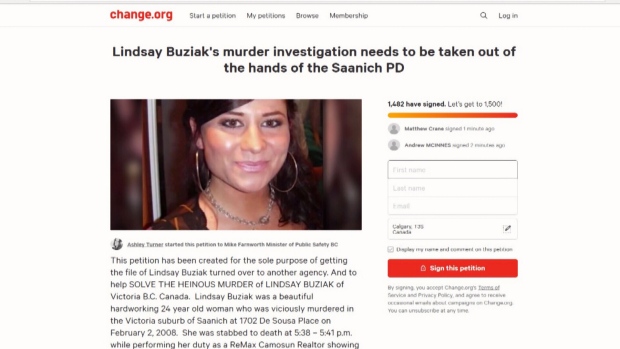This image captures a screenshot of a Change.org website displaying a petition article. The website's user interface features navigational options, including "Start a Petition," "My Petitions," "Browse," and "Membership" along the top, with a search magnifying glass icon and login option on the right.

The petition headline reads, "Lindsey Buziak's murder investigation needs to be taken out of the hands of the Saanich PD." The main body of the text elaborates that the petition aims to transfer the investigation of Lindsey Buziak's murder to another agency to seek justice for the tragic crime. Lindsey Buziak, a dedicated 24-year-old realtor from Victoria, British Columbia, Canada, was brutally murdered on February 2, 2008, while showing a property at 1702 De Sousa Place in the Saanich suburb. The heinous crime occurred between 5:38 and 5:41 p.m. Lindsey was working under the RE/MAX real estate agency at the time.

Adjacent to the article on the right, the image shows the number of petition signatures collected so far, along with a list of signatory names. Below this section, there is an area for new signers to fill out their information and a prominent "Sign this Petition" button to submit their support.